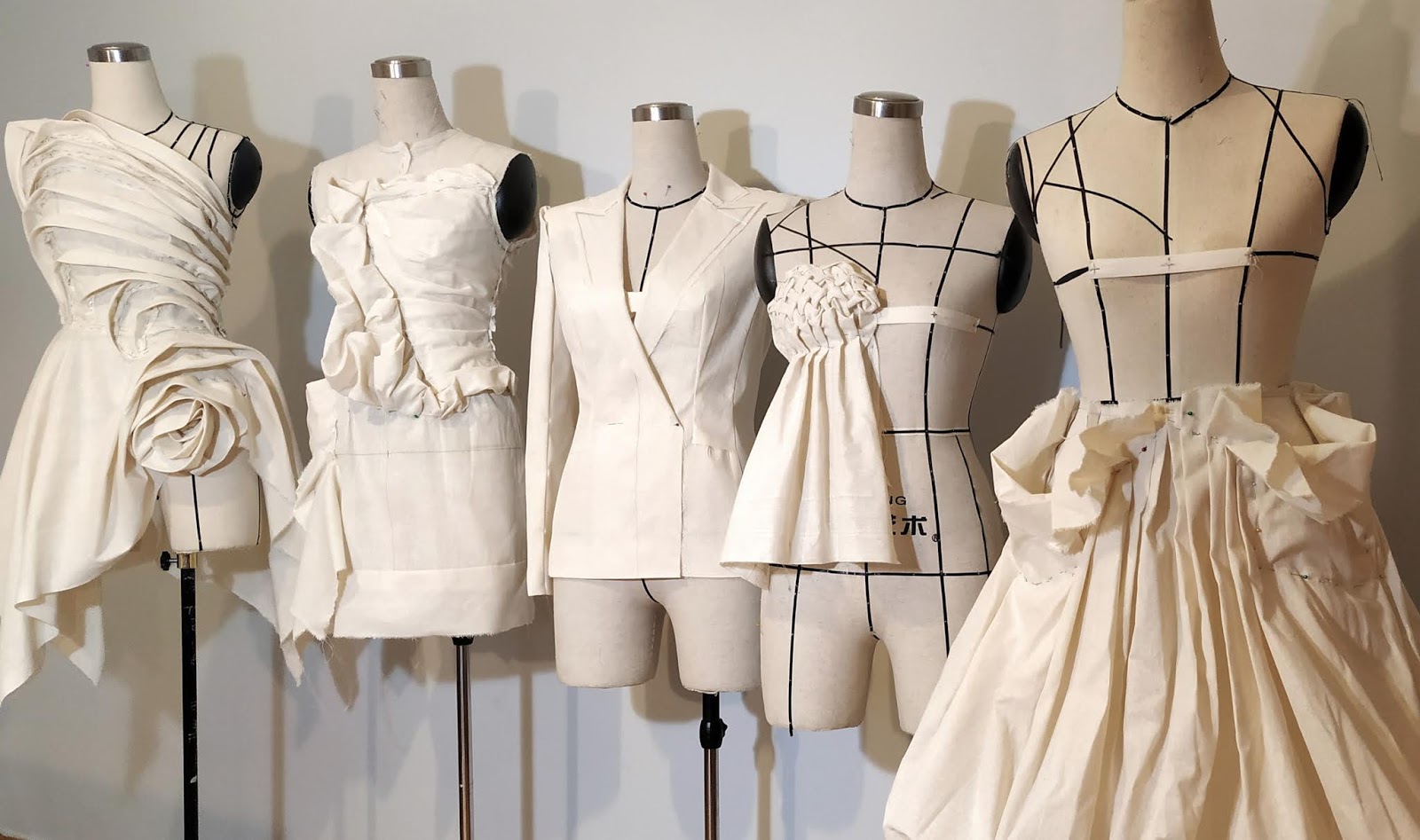This photograph showcases five half-body mannequins, all positioned in front of a beige wall. From left to right, the mannequins display a variety of neutral bridal and formal attire, suspended on poles. The first mannequin features an off-the-shoulder top with a sweeping design and a large floral detail. The second mannequin is dressed in a short ruffled dress. The third mannequin stands out with a professional casual ensemble featuring a suit jacket. Following that, the fourth mannequin wears a minimalist one-sided ruffle that drapes over part of its chest, resembling a strapless blouse. The fifth and final mannequin is adorned with a voluminous, ruffled beige skirt without any accompanying top. These mannequins are headless and armless, focusing attention solely on the detailed clothing segments.